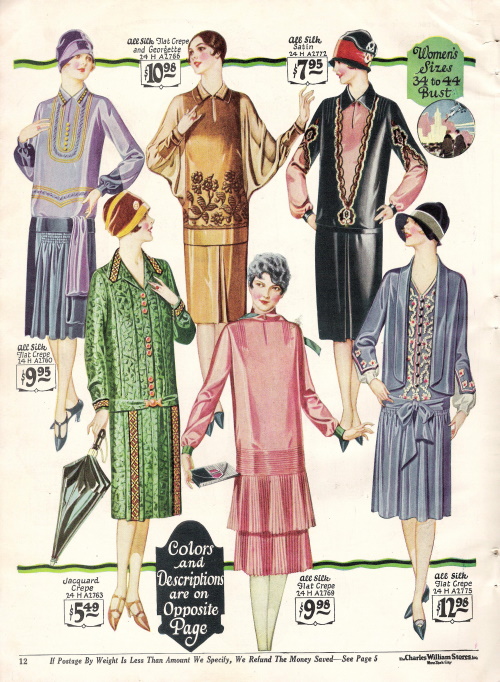This detailed and vibrant advertisement, likely from a vintage magazine or newspaper dating back to the 1950s or 60s, is a striking hand-drawn depiction of various women's clothing styles. The beautifully illustrated ad occupies page 12 of the publication and promotes elegant women's fashion with prices ranging from $7.95 to $10.98. Highlighted within the ad are garments available in sizes 34 to 44 bust, featuring an array of colors and descriptions that are referenced on an opposite, unseen page. 

The background of the ad boasts a cream color adorned with black and green wavy patterns. Five stylishly dressed women showcase the diverse outfits. One woman wears a purple dress with yellow and turquoise blue stripes paired with black heels and a 50s-style hat adorned with a small flower, priced at $9.95. Another model features slicked-back hair with a curl framing her face, donning a brown dress with sheer, lacy sleeves and brown floral patterns, and a black and red hat.

Further down, a lady in a green dress with a floral pattern is seen holding a black umbrella. Another model is dressed in a pink pleated dress, and a different figure wears a blue dress with light blue sheer sleeves and a pleated skirt, complemented by a bow around her waist. At the bottom of the ad, it reassures potential customers that any postage savings will be refunded, directing them to see page 5 for more information.